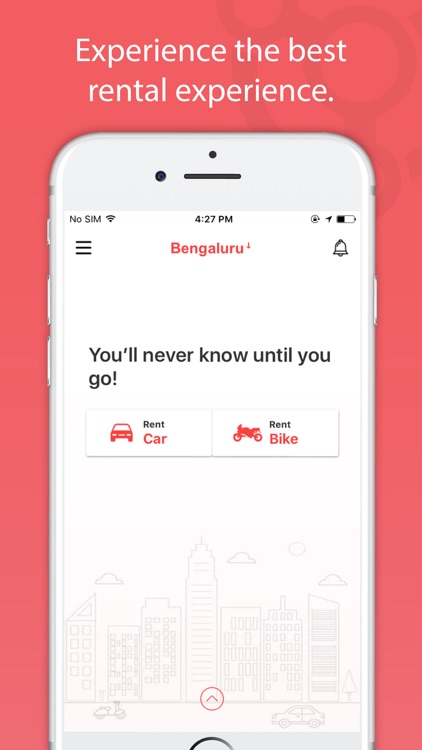A striking advertisement set against a vibrant red background showcases a sleek white iPhone, highlighting its use as a rental service tool. Subtle, darker red circles accentuate the upper right corner of the backdrop, adding a dynamic touch to the overall design. Prominently positioned at the top of the ad is a bold, white slogan proclaiming, "Experience the Best Rental Experience."

Beneath the slogan, the white-framed iPhone commands attention. At the top of the phone, a distinct horizontal slit is flanked by two small dots, indicative of the device's sophisticated sensor system. The screen displays a webpage from a site called Bingaluru, suggesting the time as 4:27 p.m. The website teases with a tagline, "You'll never know until you go," encapsulating the spirit of adventure and spontaneity.

The Bingaluru website interface offers two primary action buttons for users: "Rent a Car" accompanied by an icon of a red car, and "Rent a Bike" illustrated with a red bike. These options are neatly positioned to encourage quick decision-making for potential renters. Additionally, a menu button on the top left and an account button on the top right of the screen provide easy navigation and access to user accounts, completing the intuitive layout of the rental service platform.